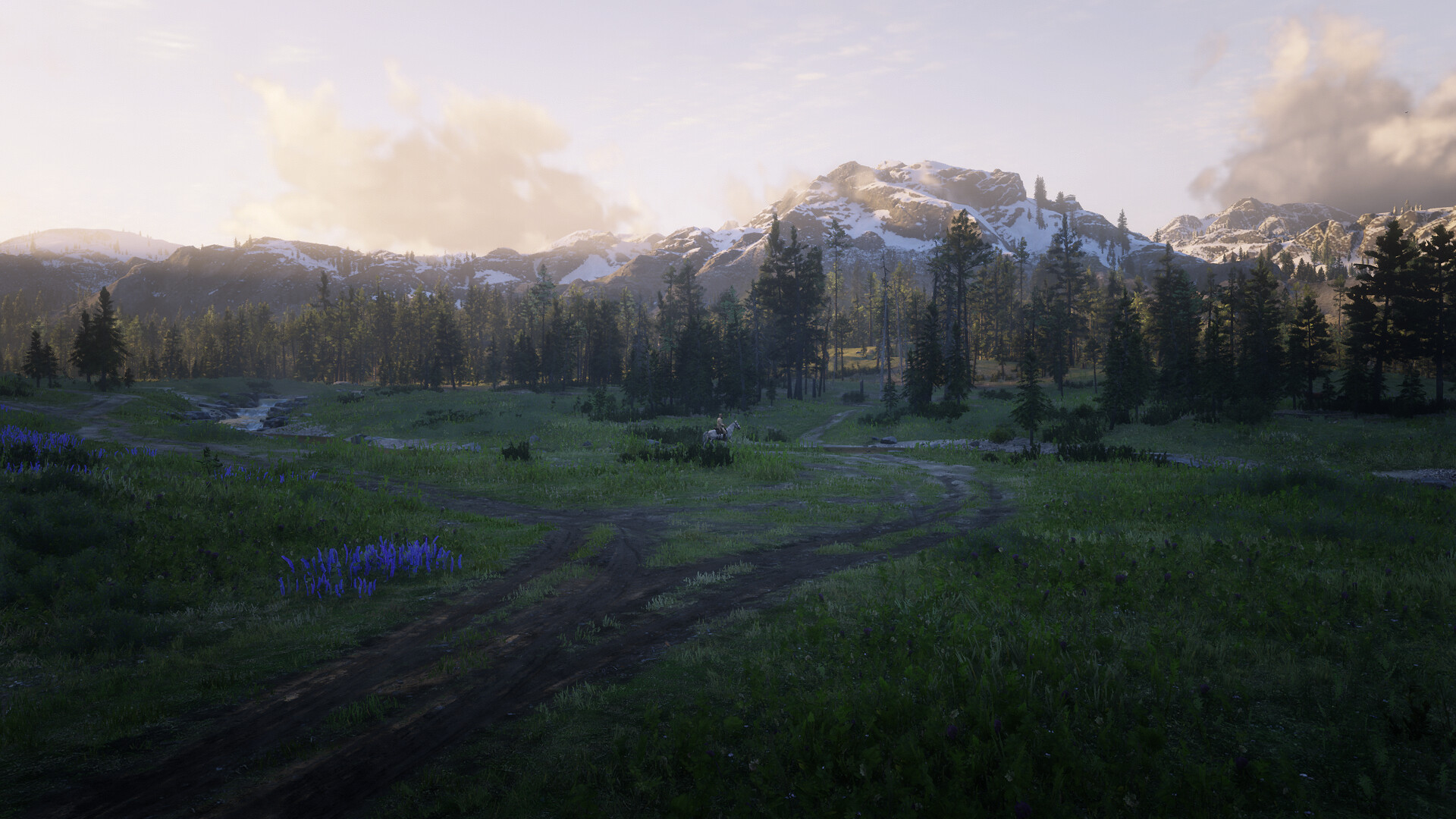A computer-generated image showcases a serene nature scene featuring a range of short, snow-capped mountains in the background. A distinct curved line of tall pine trees follows the undulating terrain, with intermittent gaps that prevent the area from appearing densely forested. In the foreground, a grassy expanse is dotted with small pools of collected water. The backdrop is a grayish-blue sky, adorned with multiple clouds clustered on the right and left sides, adding depth and atmosphere to the landscape.